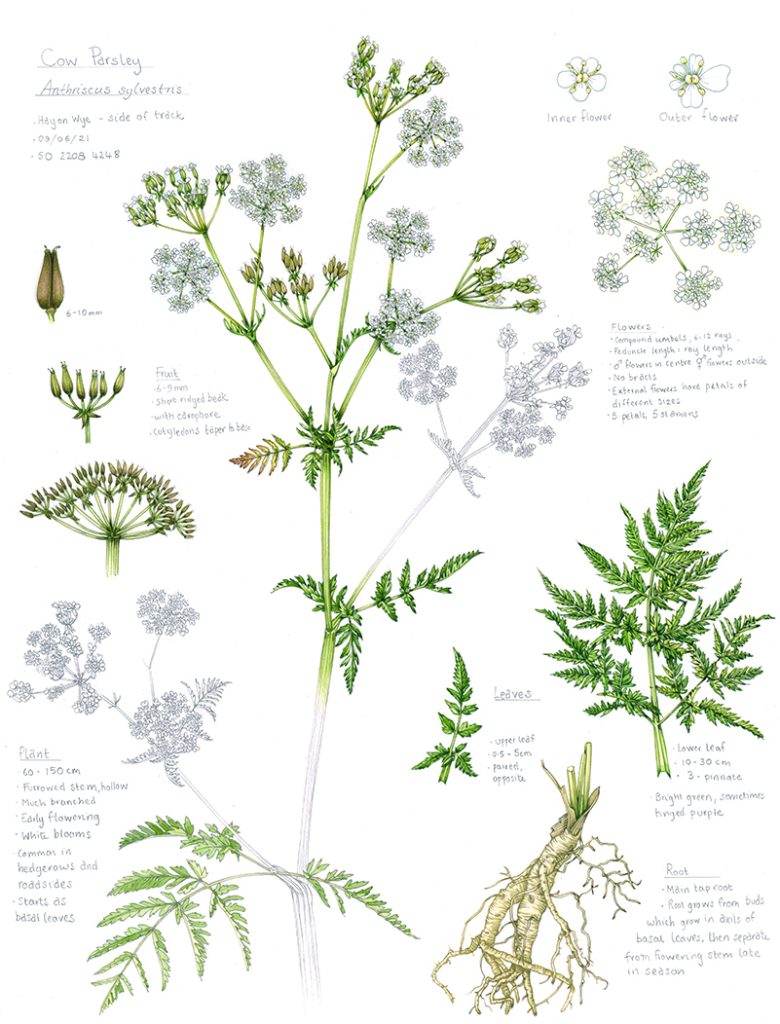This detailed illustration depicts various botanical features of the Cow Parsley (Anthriscus sylvestris) plant, rendered on a white background in portrait orientation, resembling a botanical card. The top left corner prominently displays the plant's common name "Cow Parsley" along with its Latin name "Anthriscus sylvestris," and additional text "H-E-Y-E-N-W-Y-E, side of track, 9-6-21, date," accompanied by numerical codes "50-2-2-0-8-4-2-4-8." The plant's height ranges from 60 to 150 centimeters. This detailed diagram features multiple leaf types in green and gray, with annotations specifying different parts of the plant including detailed labels for the “roots,” “leaves,” “inner flower,” and “outer flower.” The inner flower is shown with five white petals and seeds, while the outer flower has four petals, with one on the right being notably larger. Each part of the Cow Parsley is meticulously labeled and described, providing an all-encompassing depiction of the plant's structure and characteristics.